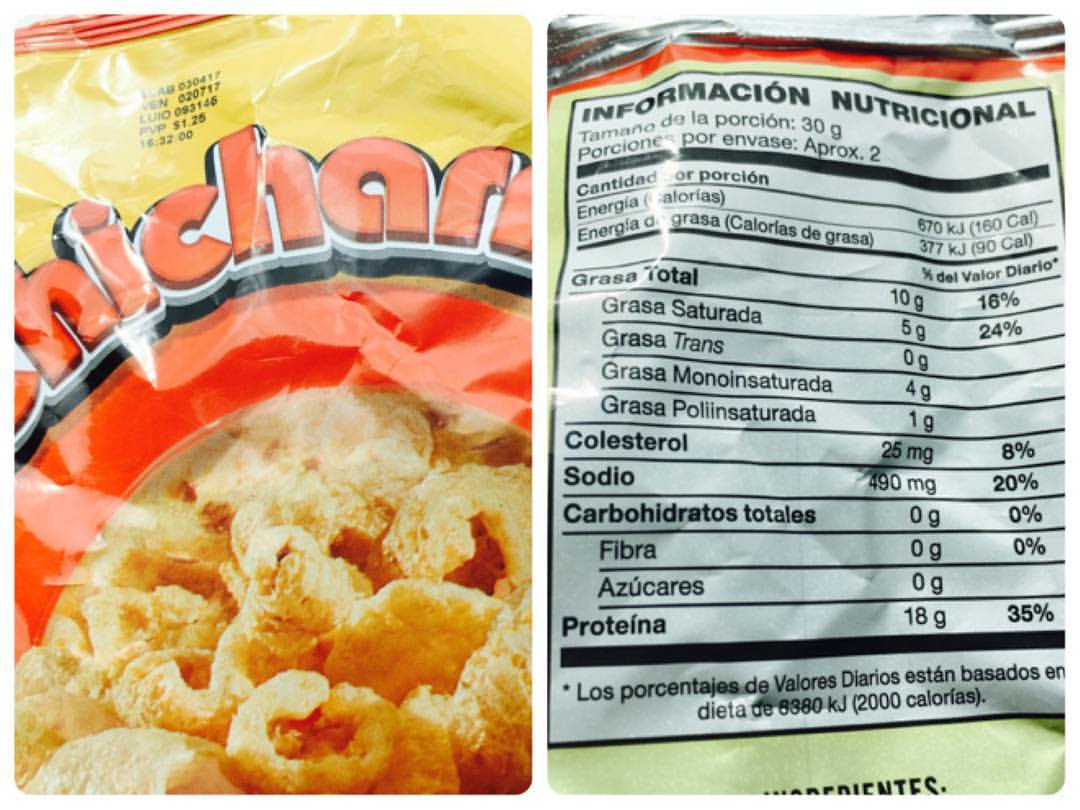This photograph features two side-by-side images of a bag of chicharrones, a popular Mexican snack. The left image shows the front of the bag, which is predominantly yellow with an orange top and border. Visible on the bag is part of the brand name, "HICHAR," in bold orange letters edged in white, along with a tempting picture of the golden, puffy, curled pork rinds. The right image displays the back of the bag, highlighting the nutritional information which is presented entirely in Spanish. At the top, it reads "INFORMACION NUTRICIONAL," followed by serving size details: "TAMANO DE LA PORCIÓN: 30 gramos" and "porciones por envase: aproximadamente dos." The nutritional breakdown includes "grasa total: 10 grams," "cholesterol: 25 milligrams," "sodium: 490 milligrams," "carbohidratos totales: 0," and "proteína: 18 grams." The back image also features a distinctive silver section with an orange streak at the top.